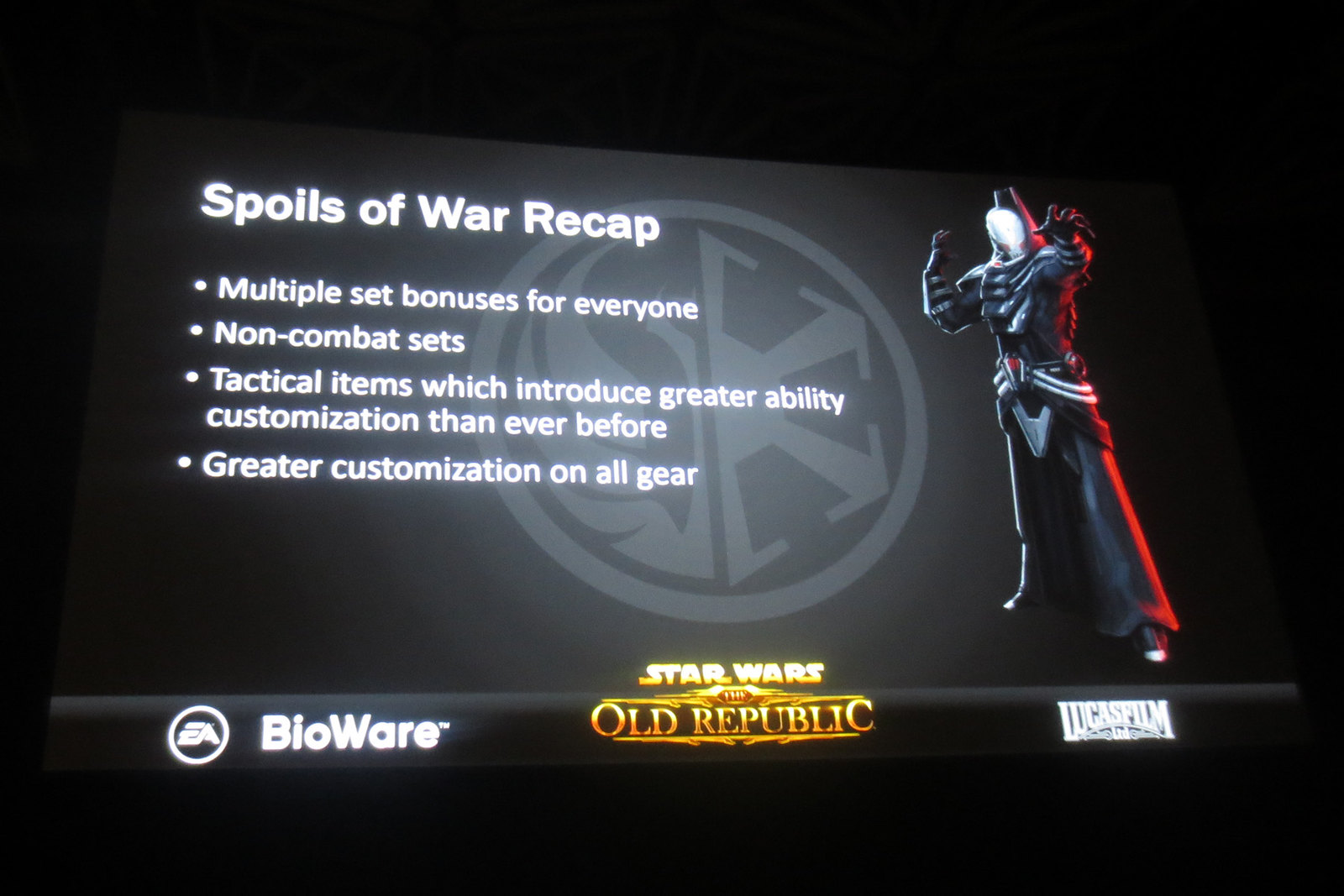The image appears to be a screen grab from a presentation or an in-game screen of the video game *Star Wars: The Old Republic*. Dominating the center-bottom of the image is the gold logo of *Star Wars: The Old Republic*, flanked by the logos of Lucasfilm Limited, EA, and BioWare. The presentation's background is black, featuring a circular gray emblem with four points and a flame-like design.

Dominating the center of the image is the title “Spoils of War Recap” in large white font. Below it, bullet points highlight features such as "Multiple set bonuses for everyone," "Non-combat sets," "Tactical items which introduce greater ability customization than ever before," and "Greater customization on all gear."

A focal point on the right side of the screen is a character from the game, draped in a dark cloak and backlit with red lighting. The character's white mask and space-age appearance add a dramatic touch, emphasizing the game's thematic depth and immersive design.